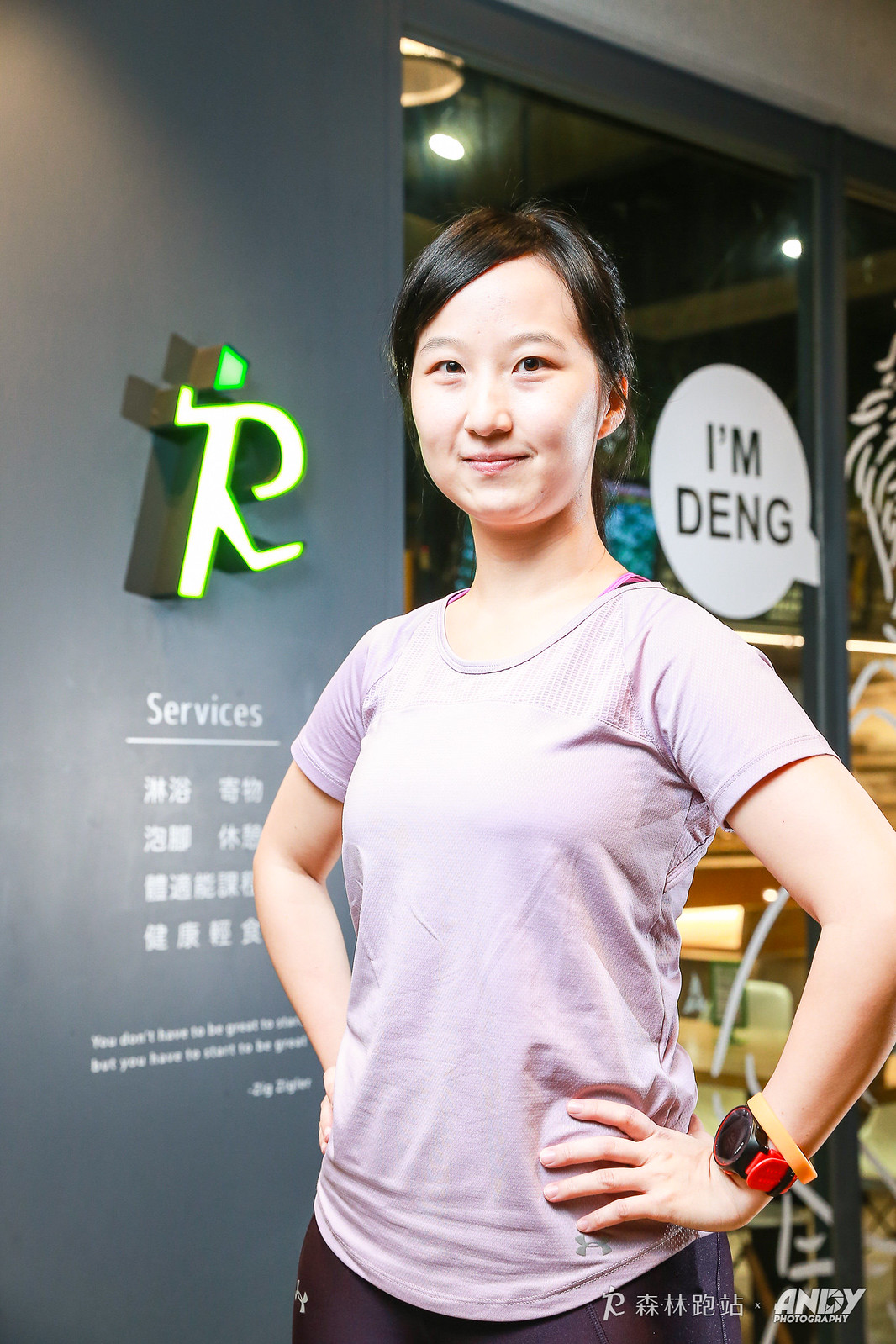This photograph captures a young Asian woman standing confidently with her hands on her hips. She is dressed in a lavender short-sleeved t-shirt and black pants, accessorized with a watch that has a red wristband on her left arm and an orange rubber bracelet. Her medium-length black hair frames her face, where she sports a slight, pursed-lip smile. The backdrop appears to be a professional or commercial setting, featuring a gray wall with a logo resembling the letter "R" and white text including the word "services" and some Asian characters. To the right, on a glass storefront, there is a talk bubble in white with black text saying "I'm Deng," and below it, a watermark that reads "Andy Photography" with a camera shutter graphic inside the letter "D." Subtle lighting and additional background elements, such as a possible wooden bench, complete the scene, enriching the overall composition.